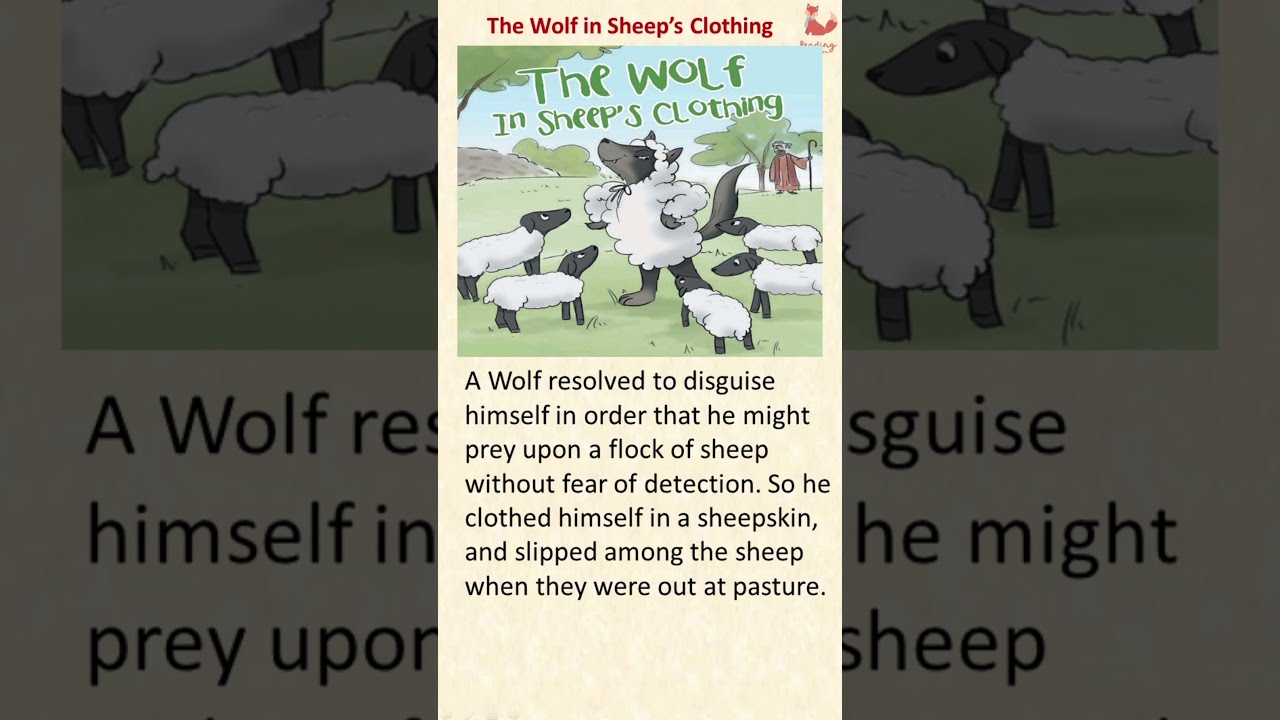The image illustrates a well-known folk tale, "The Wolf in Sheep's Clothing," and is set against a light tan background. At the top, the title "The Wolf in Sheep's Clothing" is prominently displayed in large, bold, black letters. Beneath the title lies a square-shaped cartoon illustration of several sheep standing in a grassy field. Amongst them, one sheep is conspicuously standing on its hind legs, revealing itself to be a cunning wolf dressed in sheepskin. In the background of the scene, a shepherd can be seen, seemingly unaware of the wolf amidst his flock.

Within the illustration, the phrase "The Wolf in Sheep's Clothing" is written again in green text, broken into two lines, and placed in the sky above the field. Below the illustration is a paragraph of black text that recounts the classic story: "A wolf resolved to disguise himself in order that he might prey upon a flock of sheep without fear of detection. So he clothed himself in a sheepskin and slipped among the sheep when they were out at pasture."

The central image is complemented by a faded and zoomed-in version of the same picture in the background, creating a layered, artistic effect. The overall composition serves to vividly explain the concept of the ancient fable in a clear, engaging manner.